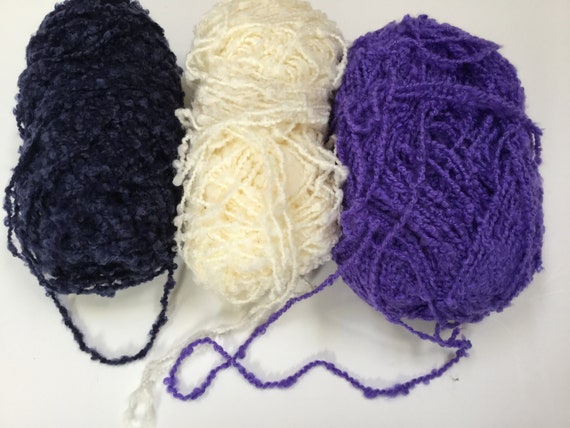The image features three balls of textured yarn, positioned in the upper two-thirds of the frame against a white background. On the left is a deep blue or black ball of yarn, loosely rolled with a noticeable texture that appears almost braided or bumpy. The middle ball is a cream or white yarn, messily wound, with its irregular strands giving it a clumpy appearance. The rightmost ball is a large, dark purple yarn, also with a textured surface. In the lower third of the frame, loose strands from these yarn balls dangle downwards, with the longest strand coming from the purple ball. The overall lighting is poor, causing the photo to appear somewhat fuzzy and out of focus, but the unique textures and colors of the yarn balls remain discernible.